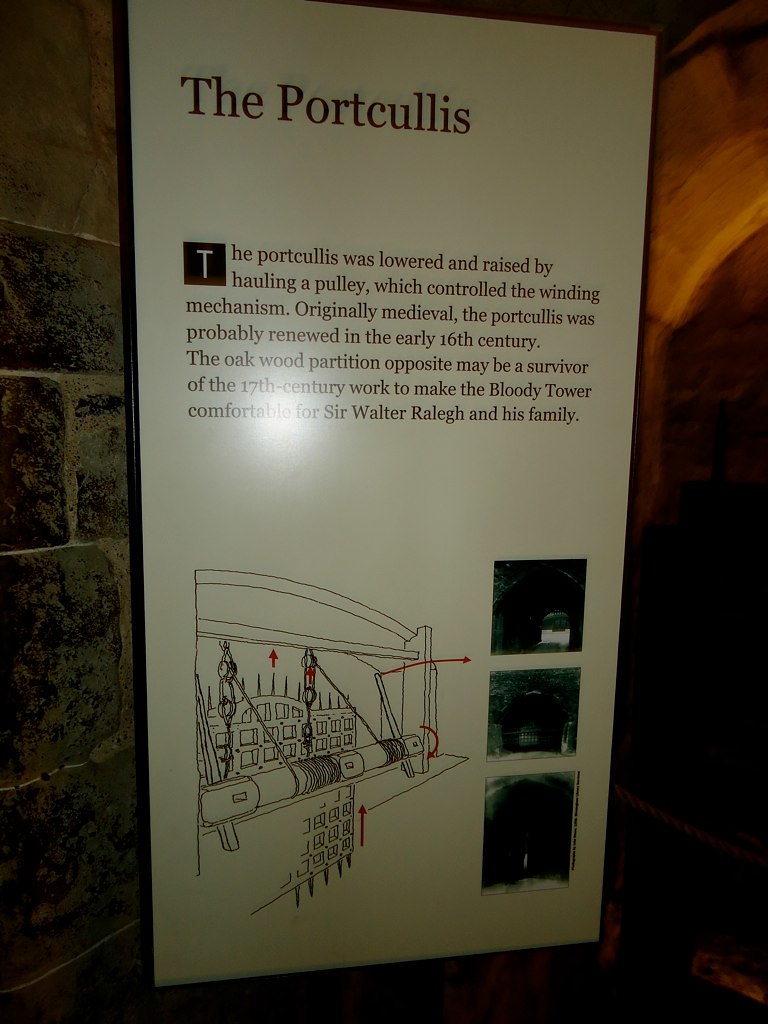The image showcases a detailed historical poster titled "The Portcullis," prominently centered against a backdrop of dark brick and stone walls. The poster features a white background framed in black, with descriptive text explaining the portcullis mechanism. It describes how the portcullis was lowered and raised using a pulley system controlling a winding mechanism, originally medieval and likely renewed in the early 16th century. The text also mentions an oakwood partition from the 17th-century renovations aimed at providing comfort for Sir Walter Raleigh and his family in the Bloody Tower. Below the text, there is a line-drawn diagram illustrating the pulley system, and to the right, there are three indiscernible dark photos. The setting is dim, with a dark cave-like hallway visible on the right, emphasizing the historical and somewhat somber atmosphere surrounding the poster.